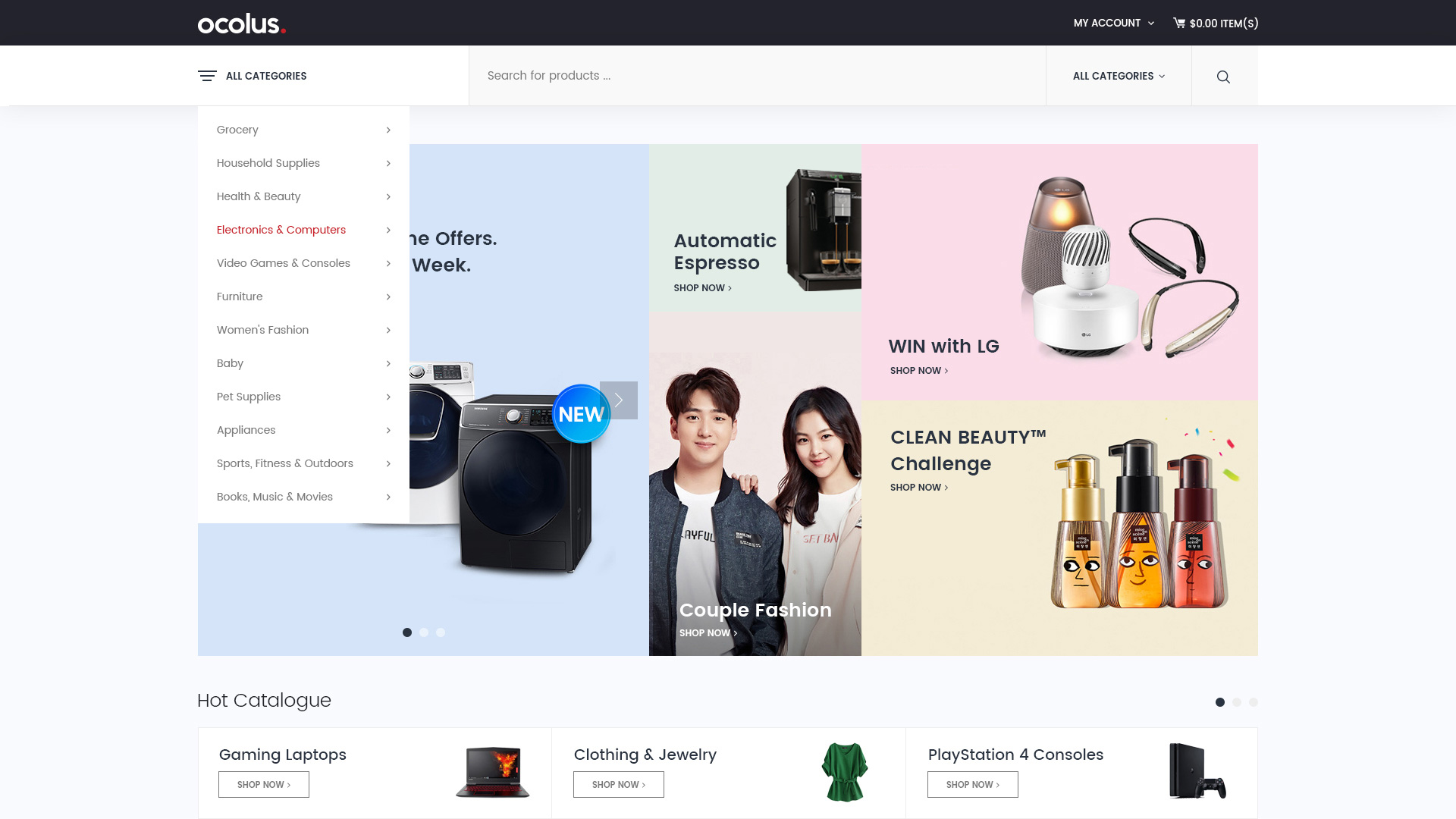The image features a user interface of an online shopping platform. At the top, there's a black rectangle with white text displaying "Oculus." Nearby, there are icons for "My Account" and a shopping cart, which indicates that there are zero items totaling zero dollars.

On the left side, a column categorizes the products with headings such as: Grocery, Household Supplies, Health and Beauty, Electronics & Computers, Video Games & Consoles, Furniture, Women's Fashion, Baby, Pet Supplies, Appliances, Sportswear, Soft Toys, Books, and Movies. A blue square background shows an image of a washing machine labeled "Poly Mag Espresso." In the center of the display, there's an image of a person dressed in a pink jacket, labeled under "Couple of Questions." 

At the top right corner, a pink square is depicted with what appears to be headphones, captioned “LG Shop Now,” promoting the "Clean Beauty Challenge."

On the bottom right, three pump bottles are illustrated with cartoon faces on their labels. The bottom left contains a banner for the "Hot Catalog," promoting items like a game laptop with a "Shop Now" button, and clothing and jewelry, specifically featuring a green shirt. There's also a "PlayStation 4 Console" with an attached controller and "Shop Now" and "Subscribe" options.

Overall, this image is a blend of various promotional elements and categories, showcasing a wide array of items available for purchase on this versatile online shopping platform.